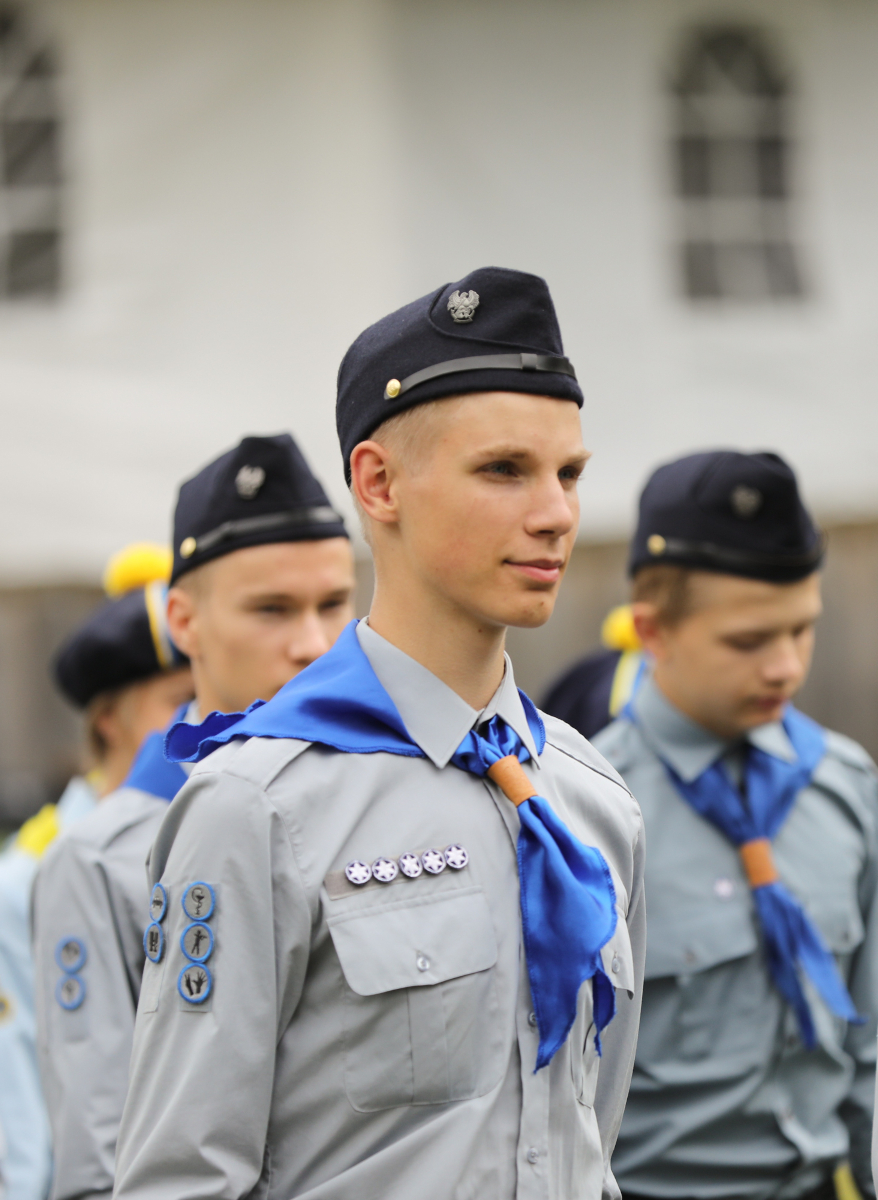The photograph shows a group of four young men, likely cadets or junior scouts, wearing nearly identical uniforms and standing at attention against the backdrop of a large white building with arched windows. All of them are visible from the waist upwards. They are dressed in gray button-up shirts with collars and two chest pockets, accessorized with blue neckerchiefs held together by small brown clasps. Each wears a flat cap adorned with a metallic badge depicting an eagle.

The young man in the forefront, who is Caucasian with short blonde hair, stands out with a slight smile on his face. His uniform is the most decorated, featuring five round badges on his right arm and five metal star badges on the left side of his chest. The individual to his right has a single star badge, while the person to his left, whose chest is not visible, displays two round badges on his arm. The navy blue hats they wear have a black strip and a gold button, further distinguished by the silver eagle emblem.

The men are positioned with a sense of order, some looking straight ahead while others gaze into the distance. Amidst them, the young man in the foreground draws the most attention, suggesting a possible rank or achievement within their group.